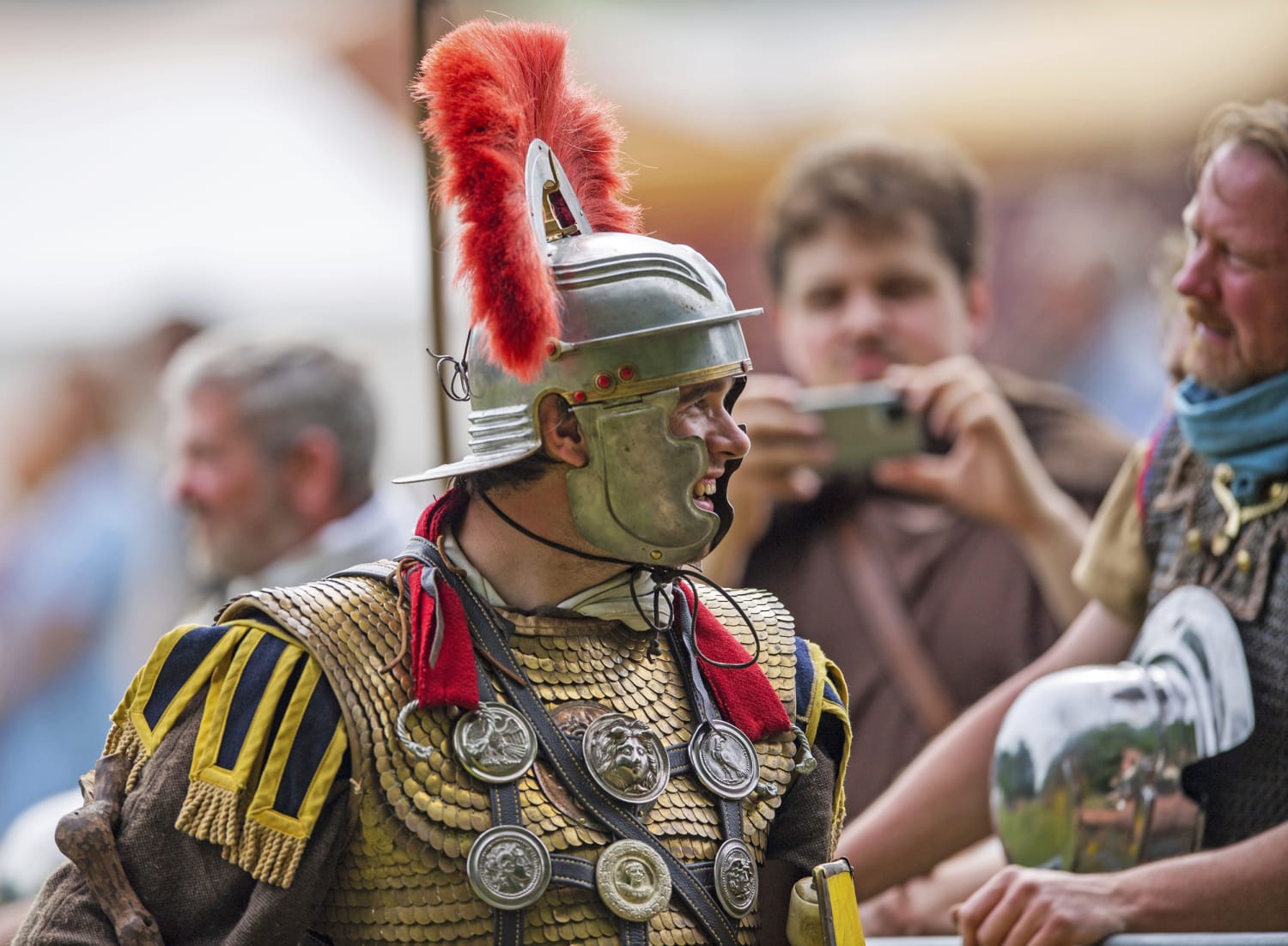This photograph captures a vivid reenactment of a Roman soldier or gladiator, focusing on a man dressed in intricate ancient military attire. The image centers on the soldier, showcasing him in a tight chest-up frame, turning his head to the right with a subtle smile. He dons a silver-colored helmet adorned with a striking red plume that arches across the top, with metal guards cascading down to shield the sides of his face.

The soldier's woven armor drapes over his shoulders and chest, embellished with various metal medals and leather straps. A red scarf-like fabric is wrapped around his neck, complemented by blue and yellow epaulettes on his shoulders. His outfit includes a rope-like vest and a belted arrangement displaying several gold coins.

In the blurred background, three people add context to the reenactment scene. One individual, dressed in a similar woven armor but without a helmet, stands to the right holding his helmet against his chest. Another person, in a brown t-shirt, captures the moment with a digital camera, enhancing the authenticity of the reenactment setting. A third person is also visible, adding to the sense of historical immersion and engagement in the event.